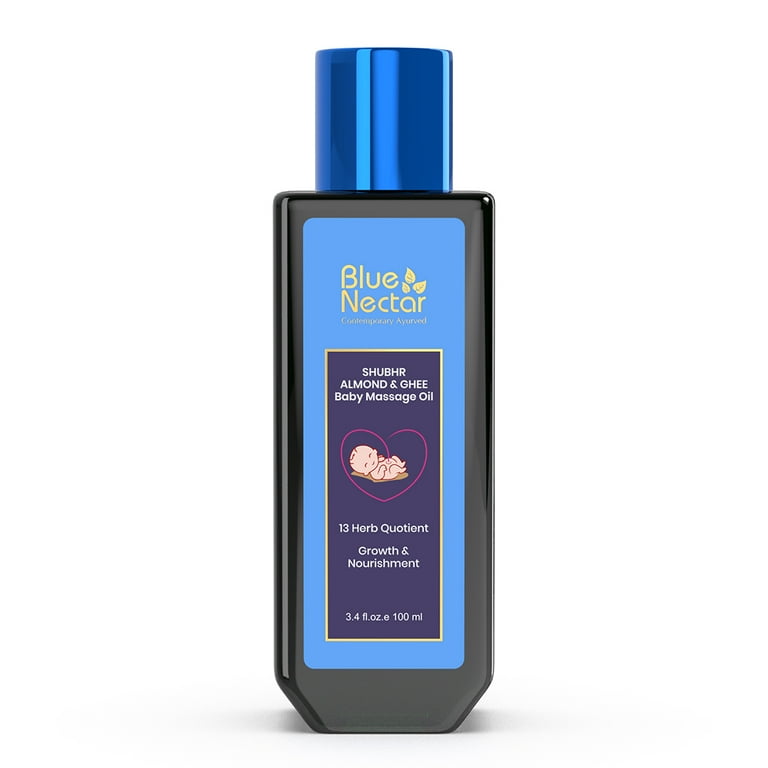The image features a dark gray, oblong, shiny bottle set against a featureless white background with subtle gray, computer-generated shading underneath. The bottle has a light teal rectangular label with rounded edges. The label prominently displays "Blue Nectar" in white font at the top, accompanied by yellow leaves on either side. Below this, a smaller dark blue rectangle contains the text "Shoe Beer, Almond, and Ghee Baby Massage Oil" in white font, along with a cartoon image of a baby inside a heart drawn with a red line. Further down, the label reads "13 Herb Quotient Growth and Nourishment," and specifies the bottle's capacity of 3.4 fluid ounces (100 milliliters). The bottle is topped with a teal cap.